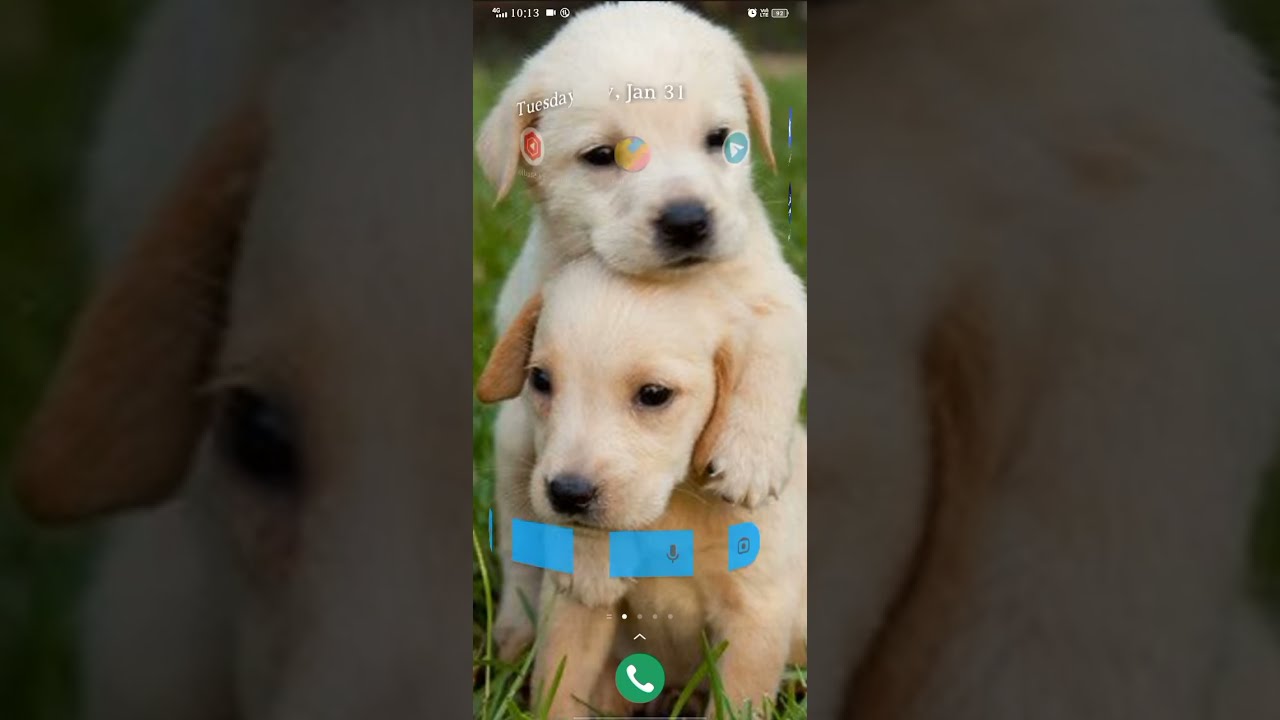The image is a detailed photograph of an Android phone screen, featuring a wallpaper of two Labrador puppies. One puppy, with a slightly lighter coat, is climbing on top of the other puppy's head, both set against a backdrop of outdoor grass. The phone screen displays critical information, indicating it was taken on Tuesday, January 31st at 10:13, with a 100% battery charge, a Wi-Fi signal at 3 bars, and a connection to a 4G network. The screen also shows an alarm icon and a small recording icon at the top. At the bottom of the screen, there's a blue call button with a white arrow pointing up. The image itself has been darkened and expanded to create a background effect, emphasizing the central portion where the puppies are featured.